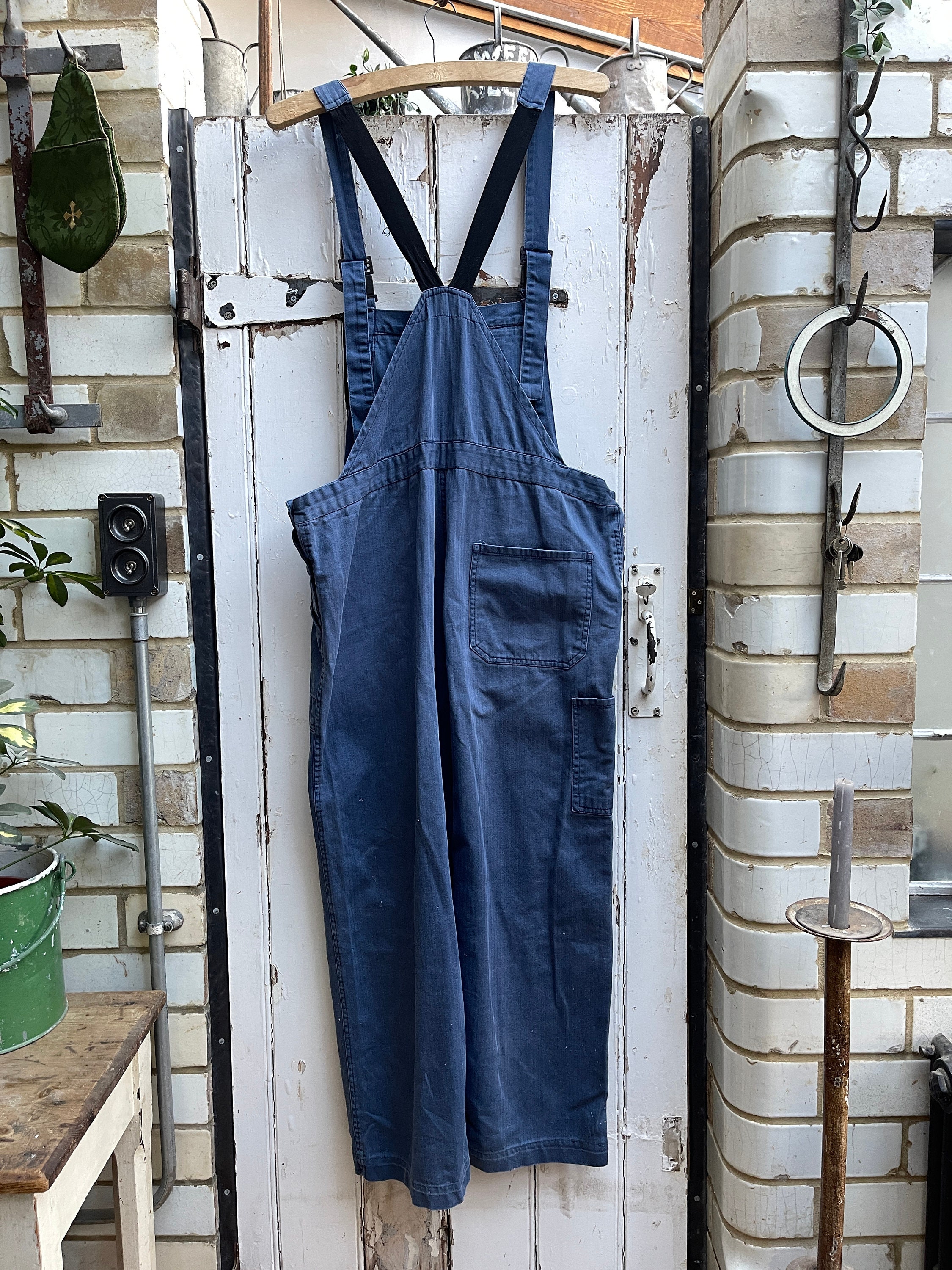The photograph captures a pair of blue overalls or a smock hanging prominently on a wooden hanger in front of a weathered, white-painted door that has seen better days, with its chipped paint and aged appearance. The setting appears to be an outdoor workshop or garden shed, due to the abundant natural light and absence of a visible roof. Flanking the door are brick walls, hosting various steel hooks and hangers. These hooks bear an assortment of gardening tools and objects, such as a ring, a satchel, and a set of keys. To the left, partially visible, is a wooden table used for potting plants, adorned with a pot from which green leaves sprout. Above the door, several watering cans are stored, reinforcing the impression of a functional gardening space. The overall scene is a blend of white, brown, and beige tones, adding to its rustic charm.